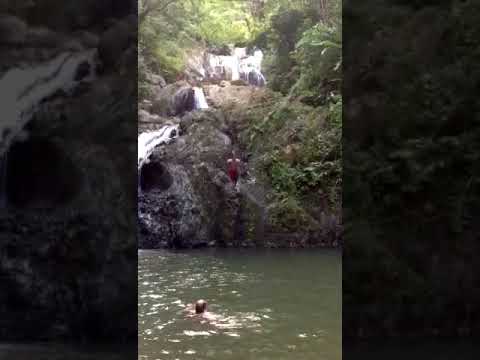In this small, low-quality photograph, we see a serene outdoor setting featuring a waterfall cascading down a rocky, cliff-like terrain into a lagoon. The water exhibits a brownish, slightly green hue. The waterfall begins at the top center of the image and flows down to the left, threading through a lush landscape filled with trees, bushes, and verdant foliage. Towards the bottom left of the photograph, a person's head is visible just above the water, suggesting they are swimming in the lagoon. Additionally, another individual, bare-chested and wearing red shorts, stands near the center atop the rocky cliffs, possibly preparing to jump. The lighting of the scene shows a sunlit backdrop, casting a glare on the leaves and water in the higher parts of the image, while the areas closer to the water are shrouded in relative shade. The image includes a thick border on the sides, where elements from the main image have been enlarged and grayed out, adding to the overall framed appearance.